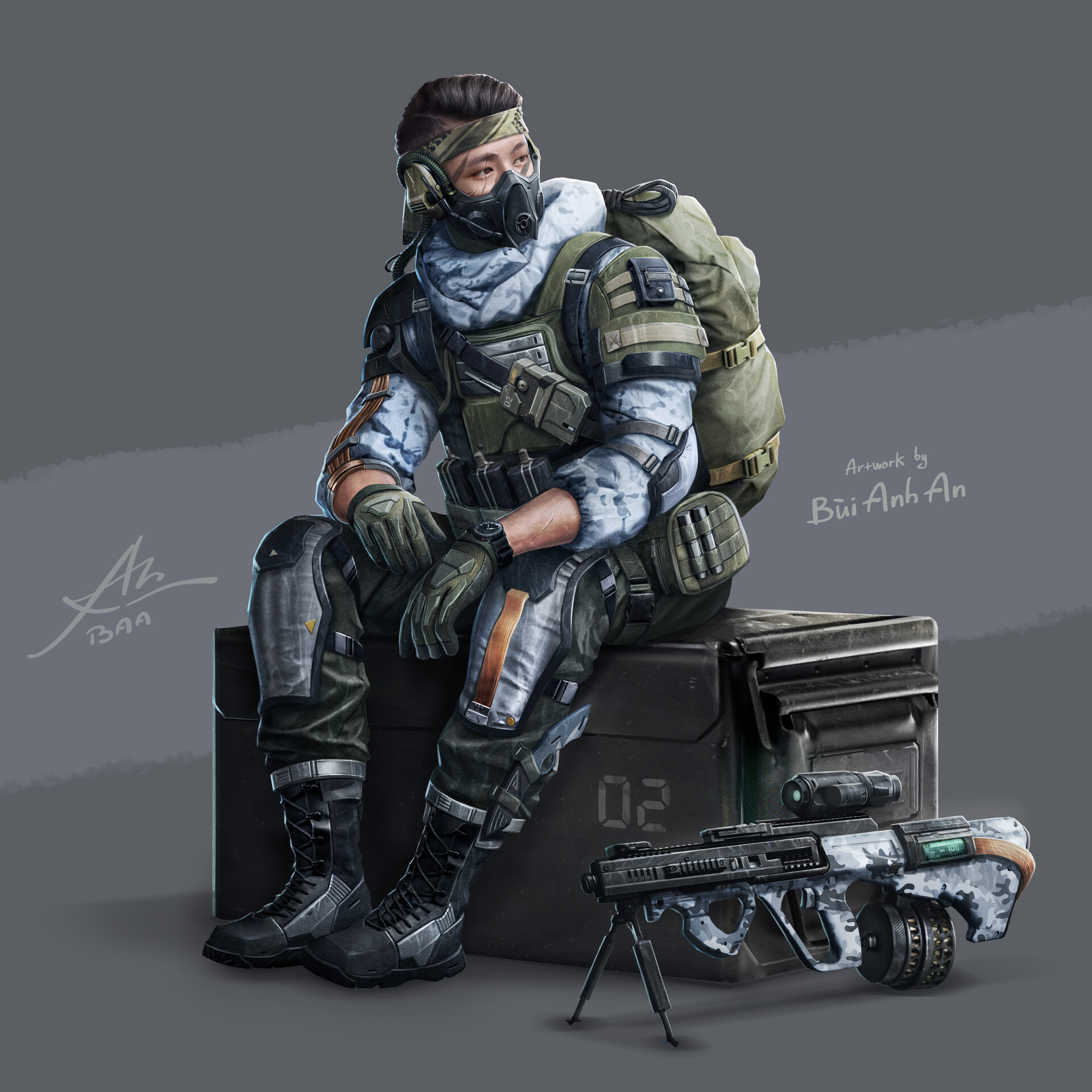This artwork is a detailed drawing of a soldier sitting on a large dark gray weapons case, used for carrying equipment such as ammunition. The background is visually segmented with various shades of gray: dark gray at the top, transitioning to lighter gray in the middle, and returning to a medium gray at the bottom. There is text on the left and right sides of the canvas, including a signature "Artwork by BUIANHAN."

The soldier, whose gender is ambiguous, is depicted with medium fair skin and dark brown hair brushed back under a green bandana. Their face is partially obscured by a black face mask. They wear a camouflage shirt with sleeves that almost reach the wrists, over which is a greenish bulletproof vest equipped with various pieces of gear. On their left wrist, there is a black watch, and their hands are gloved in dark gray.

The soldier's uniform includes military-style leggings in greenish and bluish tones, complemented by large black boots. They also carry a brown backpack. To their immediate right is a large rifle fixed on a bipod stand, positioned on the floor beside the case. This case, featuring the number "02" on its right side, has metal handles and appears robust enough to store heavy-duty equipment. The detailed portrayal accentuates the soldier's readiness and the utilitarian nature of their environment.